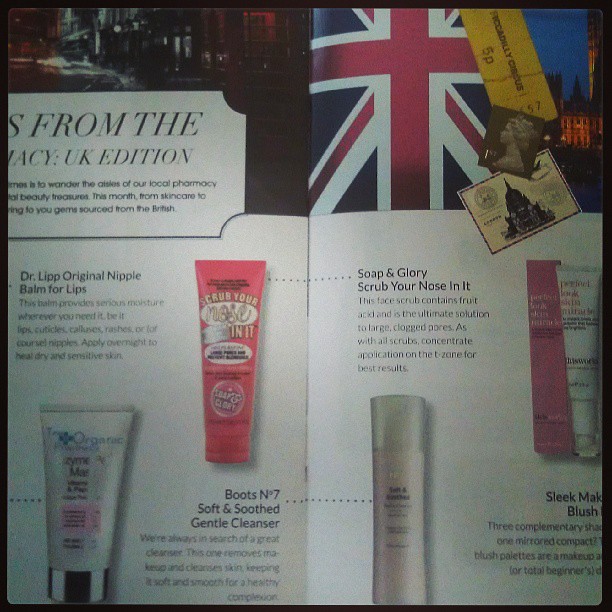This image features a magazine spread, likely from a UK beauty or product-focused magazine, showcasing a selection of skincare and beauty items. On the right page, a British flag is prominently displayed with British stamps superimposed over it. Below this, the text "Soap and Glory Scrub Your Nose In It" is visible, accompanied by a blurb that is too blurry to read. To the right of this section are two tubes of products, though their labels are unclear. Further down, the text "Sleek Make" can be discerned, followed by "Lush," with additional unreadable text due to blurriness. 

On the left page, though partially cut off, it mentions the "UK edition." Below this, the caption "Dr. Lip Original Nipple Balm for Lips" is clear, followed by another unreadable paragraph. There is a tube of product to the right of this text, which is labeled "Boots No. 7 Soft and Soothed Gentle Cleanser," and another tube to the left whose details are not readable. The spread appears to promote various creams, cleansers, moisturizers, and lip balms, aiming to cater to different skincare needs. The overall image quality is noted to be low to medium, with several parts being blurry and hard to read.